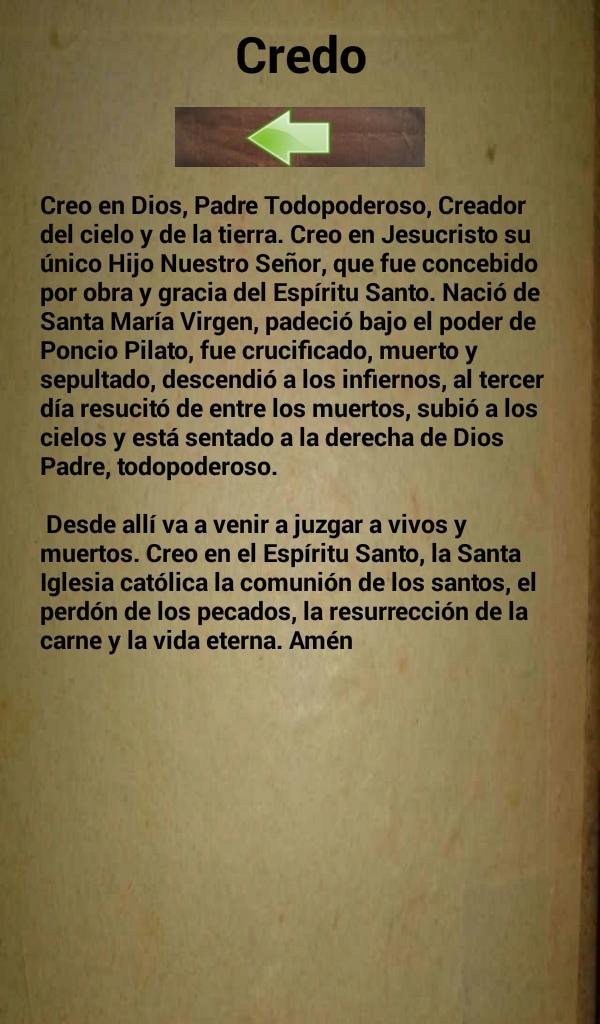The image features a rectangular placard with a faded tan, paper bag-colored background. At the top, in bold black font, is the word "Credo" with a capital 'C'. Below this, centrally positioned, is a thick green arrow pointing to the left, set within a smaller brown rectangular box. Beneath the arrow, there are two paragraphs of text appearing to be in Spanish. The content of these paragraphs resembles a prayer, with the final word being "Amen."